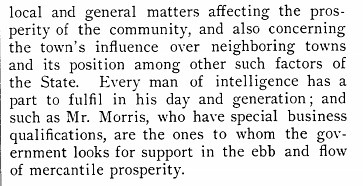The image depicts a screenshot of a paragraph of black text in a small Times New Roman font on a solid white background. This text appears to be an excerpt possibly taken from a book or newspaper article. The passage begins in the middle of a sentence and discusses local and general matters influencing the prosperity of a community, the town's impact on neighboring towns, and its broader relevance to the state. It emphasizes that intelligent men, like Mr. Morris, who possess special business qualifications, are essential to the government in navigating mercantile prosperity. The text is plain with no additional formatting, and there is a black line indicating a margin on the side. No other elements are present in the image beyond the text itself.